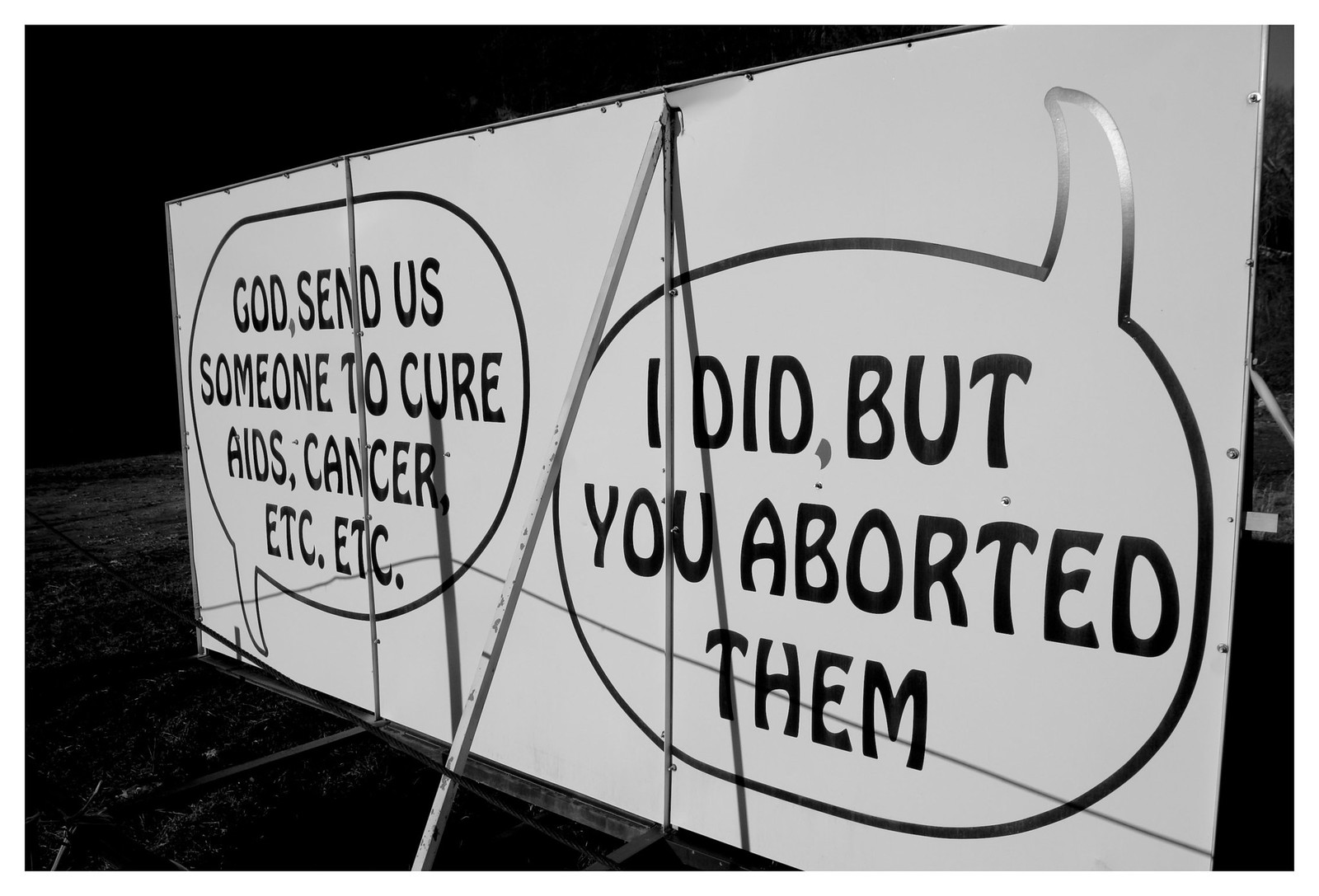The black and white image depicts a pro-life sign mounted on a white board, supported by a metal frame with visible bolts. The board features two conversation bubbles: the first, originating from the bottom, reads "God, send us someone to cure AIDS, cancer, etc., etc." The second bubble, pointing upwards, responds with "I did, but you aborted them." This anti-abortion message is starkly contrasted against the dark background, making the text more prominent. The setting appears dimly lit, possibly in the middle of a room, with a black backdrop. The metal frame holding the sign has a narrow strip of metal at the edges, and the view extends to show a line meeting the pavement and a grassy shoulder of the road in the distance.